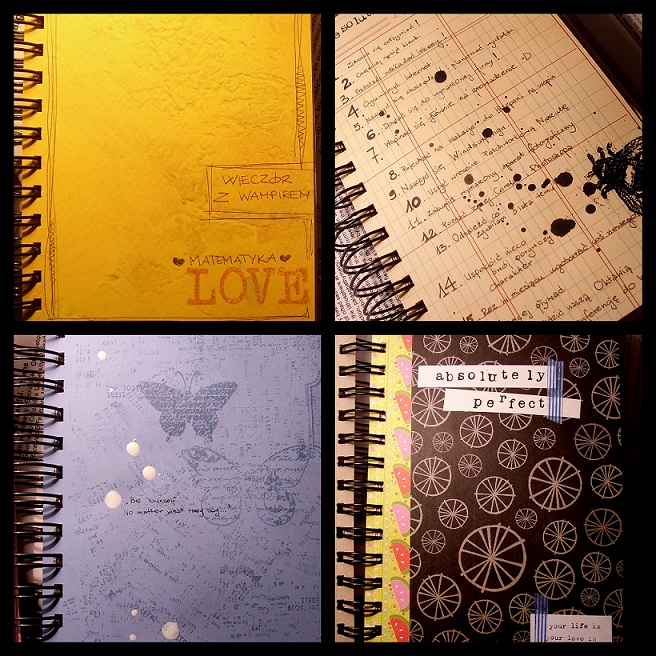The image showcases a collage of four notebooks, arranged in a 2x2 grid, each with distinctive features bound together by black wire rings. The top left notebook has a yellow cover adorned with Polish text, and in its bottom right corner, the word "love" is stamped in bold red letters. To its right, the top right notebook is open, revealing a page lined with numbers from 1 to 15, filled with written text in Polish. This page also has noticeable ink stains and a stamped image of an insect, possibly a fly or a ladybug. 

In the bottom left corner, a notebook with a blue cover features butterfly stamps and the inspirational phrase "Be Yourself" along with "No Matter What They Say." This cover includes white dots scattered across it. The bottom right notebook stands out with a mix of brown, black, and yellow-orange hues. It bears the phrase "Absolutely Perfect," accompanied by small white wheel designs and watermelon illustrations next to the bindings. The entire arrangement of notebooks is separated by black borders, creating a tidy, collage-like presentation.